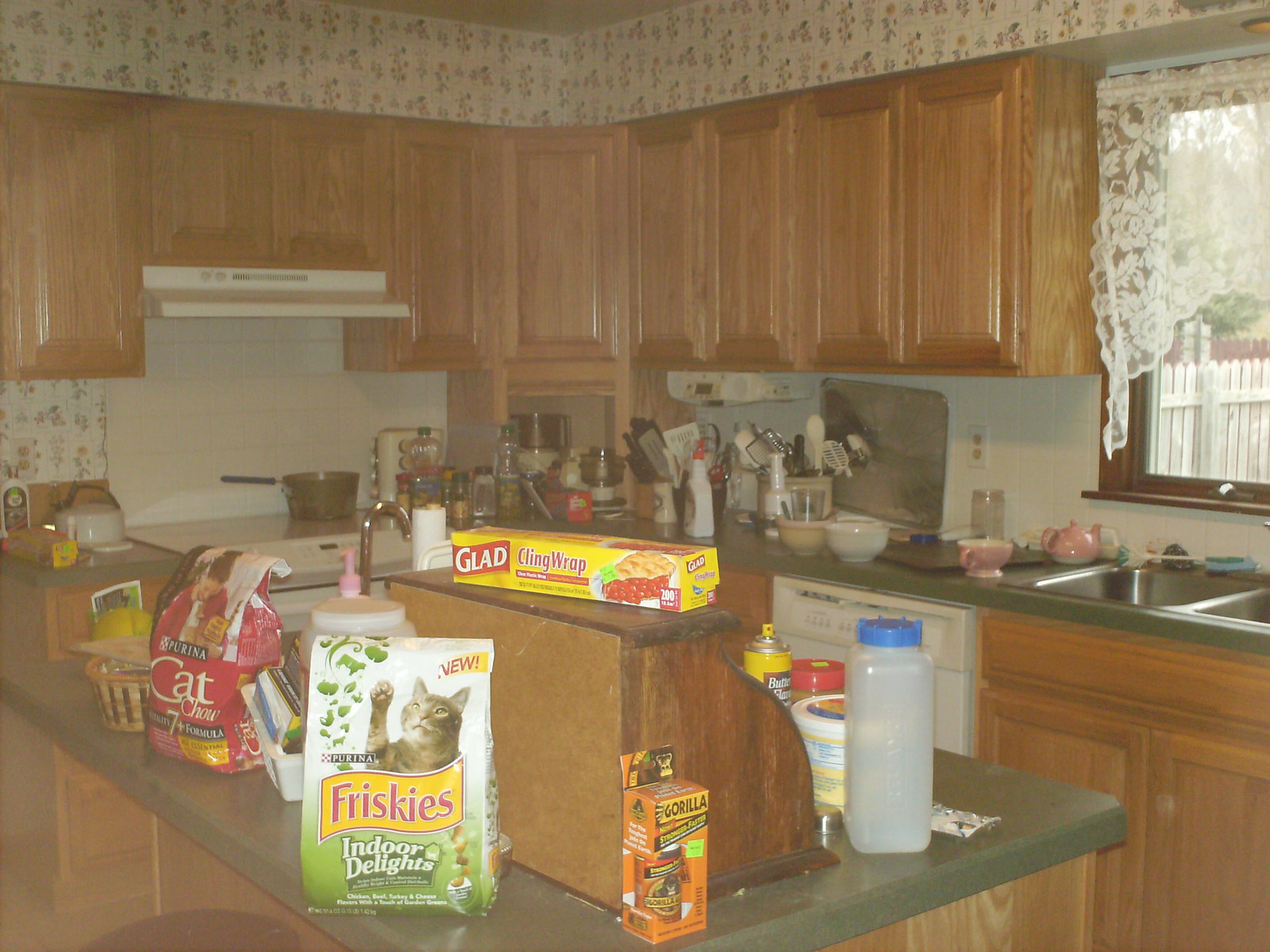The photograph depicts a cozy 1980s or 1990s kitchen, characterized by its distinctive decor and layout. The room features shiny, oak-grain wooden cabinets that lack visible handles, suggesting they are operated by recessed pulls. A white wallpaper with an indistinct but repetitive pattern adorns the walls, providing a nostalgic touch. 

The kitchen corner includes a shorter section on the left with a floor-level stove and an overhead light fixture, while the right section showcases additional cabinets. A window framed by a lacy white curtain topper sits above a stainless steel sink. The countertop below the window is a grayish-green Corian material and is cluttered with various kitchen essentials, including utensils, bowls, cutting boards, and a container holding an array of spoons.

In the foreground stands an island, crowded with numerous items such as a rounded bread box turned away from the camera, a bag of Frisky's Indoor Delights cat food, Purina cat food, a Gorilla Glue box, Glad cling wrap, a basket containing assorted objects, and a white opaque plastic bottle with a blue lid. 

Overall, the kitchen appears lived-in and functional, with a busy countertop and a slightly faded quality to the image, adding to its nostalgic charm.